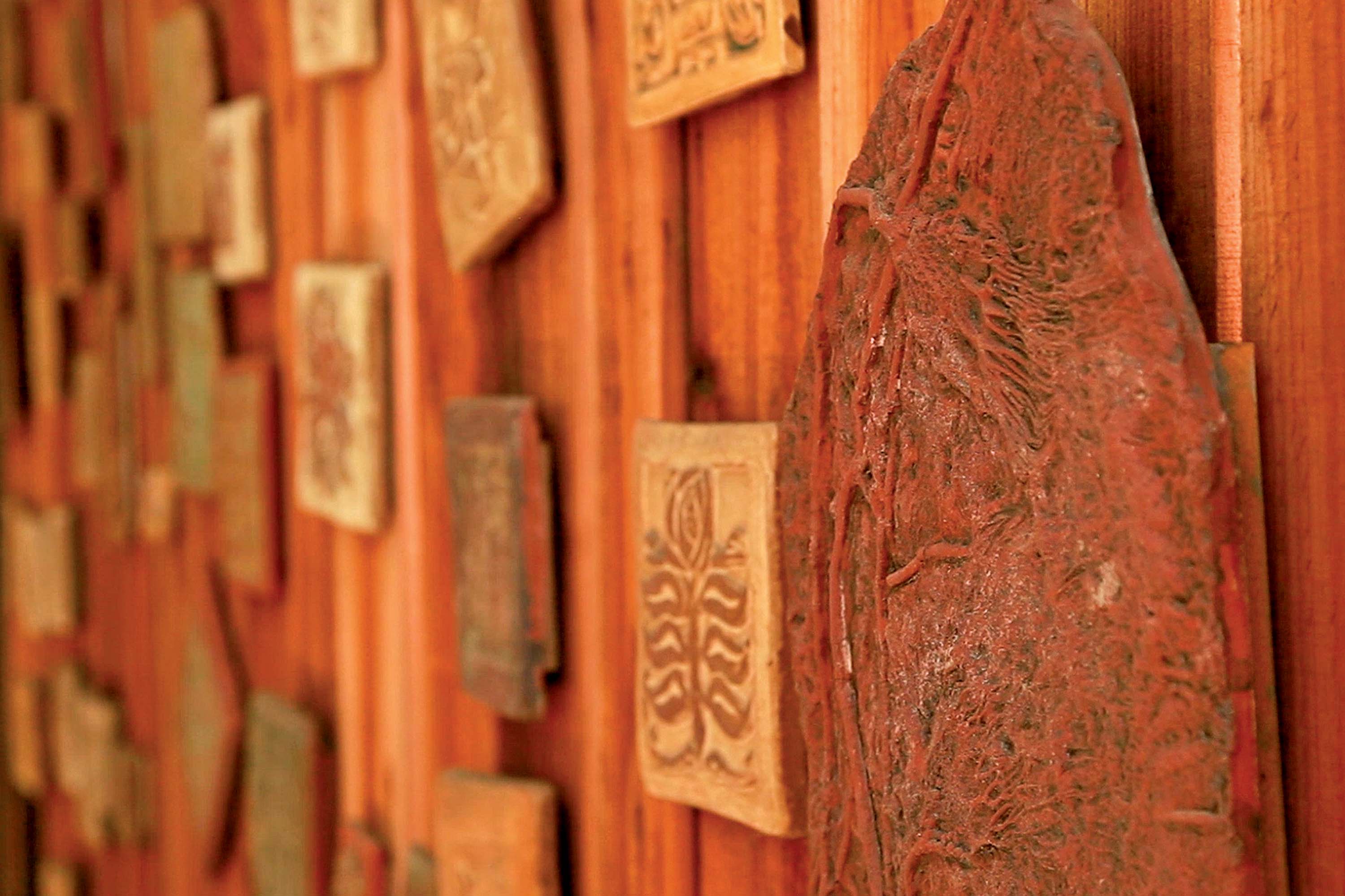The image showcases an indoor display of artwork mounted on a textured, warm-toned wooden wall. The wall features ridges, giving it a multi-dimensional feel, and the entire scene is bathed in an orange hue. The display comprises numerous small square and rectangular pieces of art that resemble ceramic or clay tiles, each adorned with rustic, outdoor-themed designs like trees, leaves, and flowers. These decorations vary in shades of orange, tan, and brown, contributing to a cohesive and earthy aesthetic.

In the foreground, a prominently visible tile exhibits a tree or leaf pattern, revealing a naive artistic style. Near this tile, an unusual sculpture draws attention—a fleshy-colored, oblong object that resembles a tongue or a sinewy peach pit. This sculpture hangs conspicuously on the wall, adding a bizarre, almost unsettling contrast to the otherwise natural-themed artwork.

The background tiles become increasingly out of focus, emphasizing the depth of field in the photograph and highlighting the details in the foreground. The scene gives the impression of being either in a cozy home setting or possibly a shop where these artistic pieces are available for purchase.